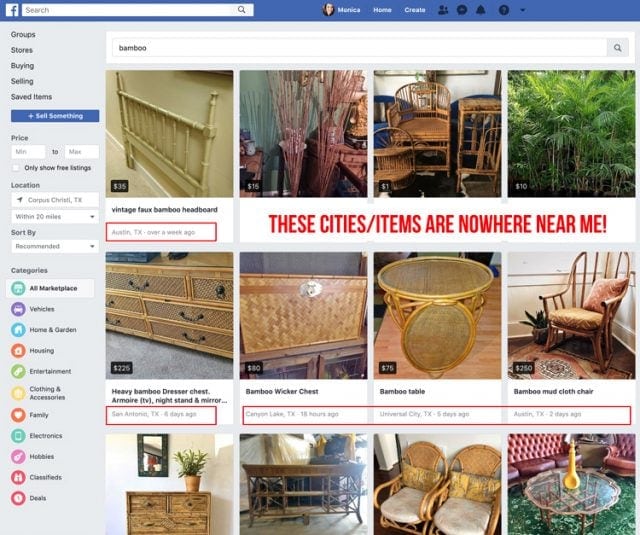This image captures a screenshot of an older version of Facebook. Along the top, there's a distinct blue bar featuring the white Facebook logo, a prominent white search bar, an indiscernible profile photo icon, various unreadable white text, and several dark blue icons. 

A sidebar on the left-hand side lists options such as Groups, Stores, Buying & Selling, and Saved Items. There’s also a prominent blue button labeled "Sell Something." Additional filtering options are included, such as price range (min to max), a checkbox for "Only Show Listings" that is currently unselected, and location filters indicating "Corpus Christi, Texas" within a 20-mile range. The sidebar also includes categories like All Marketplace (currently selected), Vehicles, Home & Garden, Housing, Entertainment, Clothing & Accessories, Family, Electronics, Hobbies, Classifieds, and Deals.

The search bar contains the term "bamboo," resulting in 12 displayed items. The top row features four images related to bamboo products. A red, all-caps text message announcing "THESE CITIES/ITEMS ARE NOWHERE NEAR ME" indicates user frustration. Red boxes outline locations such as Austin, Texas; San Antonio, Texas; Canyon Lake, Texas; Universal City, Texas; and Austin, Texas again, reinforcing the user's dissatisfaction with the proximity of the search results. This screenshot evidently aims to highlight issues with the geographical relevance of search results on the Facebook Marketplace.